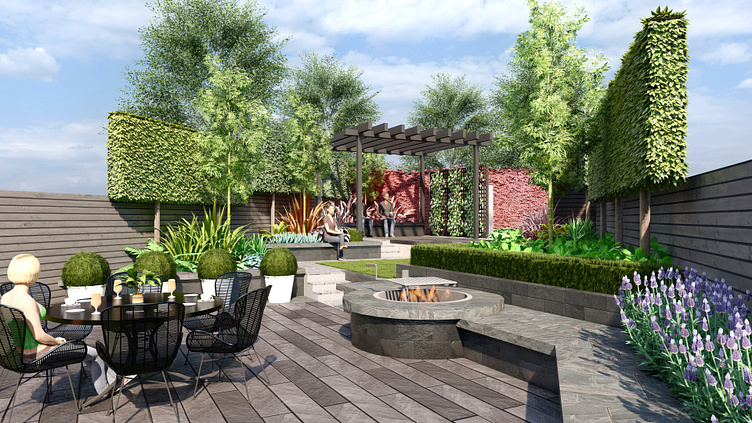The image appears to be a computer-rendered scene of an outdoor living space, possibly an architectural design for a patio area. The floor is composed of wooden planks, creating a cohesive theme along with the wooden plank walls that enclose the space. Dominating the foreground on the left is a table surrounded by six chairs, with a woman characterized by her light-colored long-legged pants and green top sitting at one of them. The table features four drinks, adding to the realistic detailing.

In the center of the space, there is a gray fire pit, flanked by benches. The backdrop includes diverse vegetation such as large trees, bushes, and small plants, as well as hedges and a brick wall extending into the far distance. Purple flowers adorn the right-hand wall, enhancing the aesthetic appeal. To the left of the scene, a man in a blazer with a red undershirt is seen walking towards the area, while a dark-brown-skinned individual is seated on a bench near the middle. Moreover, a raised section or white stairs is faintly visible in the far background.

The setting is under a partly cloudy sky, adding to the outdoor ambiance, and the entire image retains a virtual reality or artificial intelligence-generated feel, as noted by the detailed and crisp rendering style.